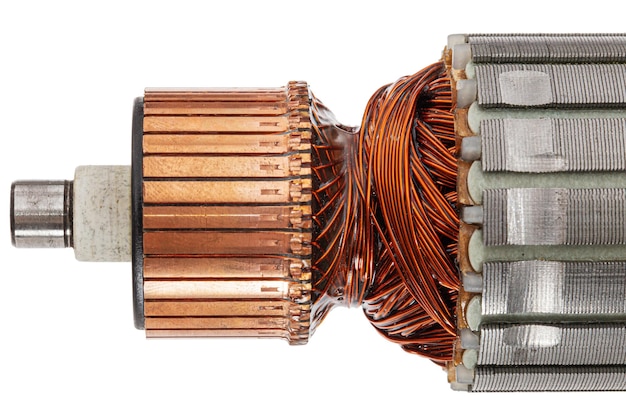This image showcases a sophisticated mechanical or electrical component set against a plain white background. The component features a distinct progression in size from left to right, beginning with a small, polished silver cap on the left. This cap attaches to a white rubber nozzle with a small silver bolt cap at its tip. Moving rightward, the nozzle connects to a smaller cylinder made of brass horizontal plates, presenting a round, smooth, and reflective surface. Further along, a convoluted array of intertwined copper wires extends from this brass portion, bending and twisting, and creating a complex network leading into a larger cylindrical attachment. This attachment consists of stacked metal rectangular plates with thin ridges and occasional beveling, extending toward the widest point on the right. The overall arrangement resembles intricate machinery parts, potentially part of an engine or an electric drill, highlighting an intricate blend of polished metals and detailed wirework.